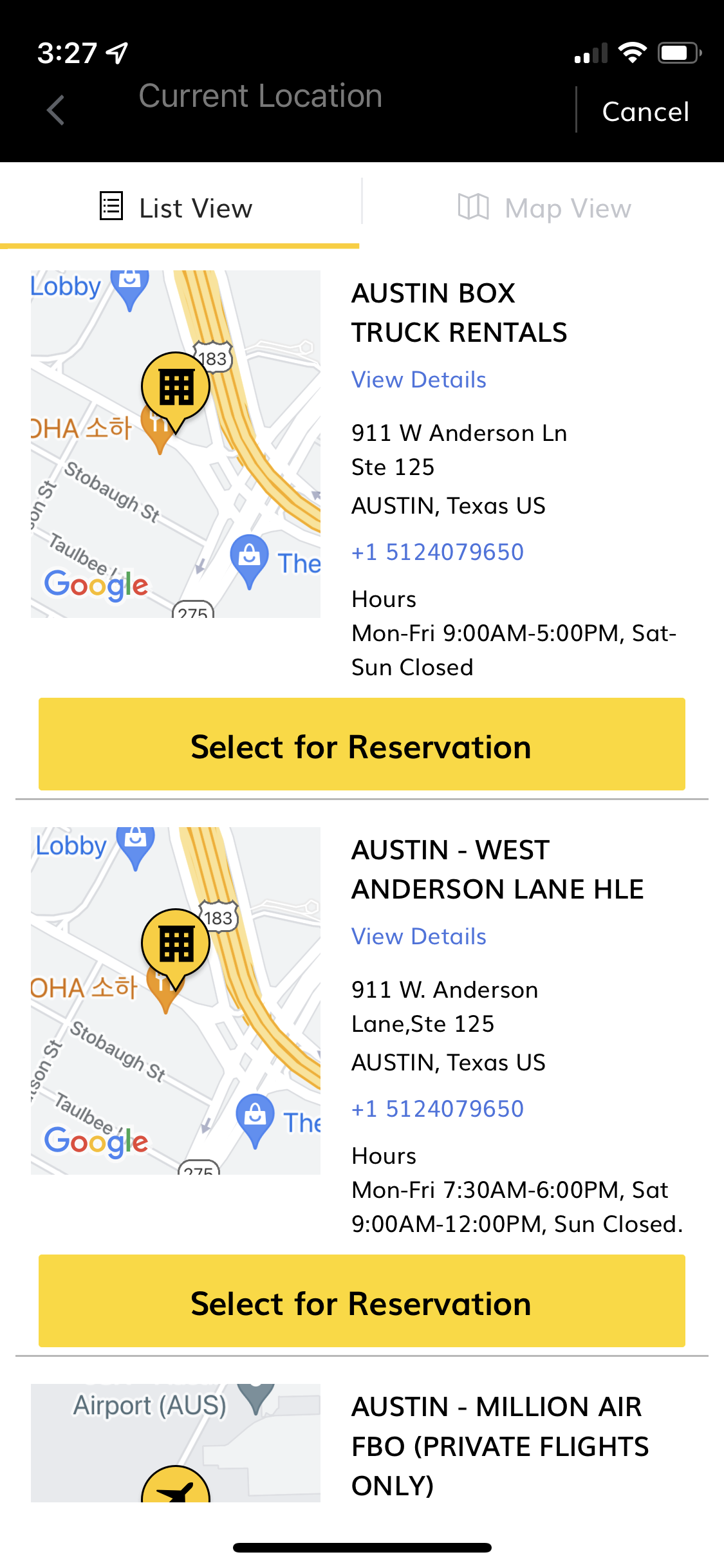A smartphone screen displaying a reservation app for box truck rentals. The status bar at the top shows cell signal bars to the left and Wi-Fi and battery indicators to the right. Below the status bar, it says "Current Location" with options for a list view and map view. The visible listings include:

1. **Austin Box Truck Rentals** - Details for this location include the address, "911 West Anderson Lane, Suite 125, Austin, Texas." Contact number: "(512) 407-9650". Operating hours: Monday to Friday from 9 a.m. to 5 p.m., Closed on Saturday and Sunday. There is a blue "View Details" link and a prominent yellow "Select for Reservation" button.

2. **Austin West Anderson Lane HLE** - Details for this location also include the same address, "911 West Anderson Lane, Suite 125, Austin, Texas," and the same contact number: "(512) 407-9650". Operating hours are listed as Monday to Friday from 7:30 a.m. to 6 p.m., Saturday from 9 a.m. to 12 p.m., and Closed on Sunday. Like the first listing, this also has a blue "View Details" link and a noticeable yellow "Select for Reservation" button.

The map on the side features various colors including gray, blue, yellow, red, and green, highlighting different areas and routes.